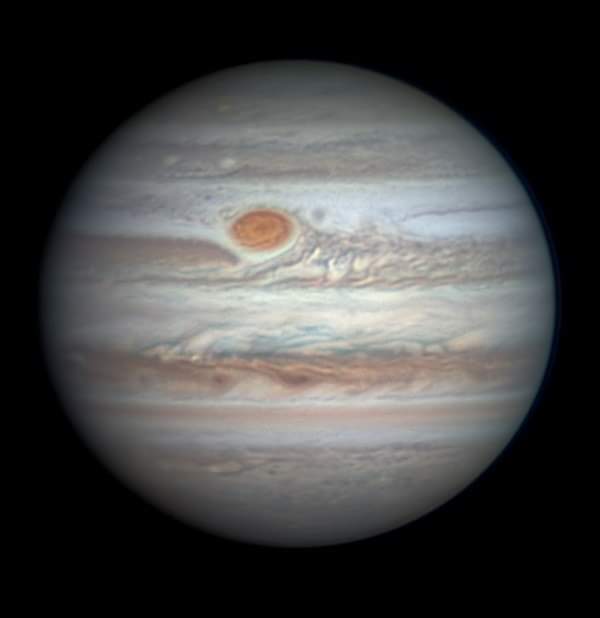The image is a close-up, square photograph of a planet set against a pure black background. Dominating the center of the frame, the planet is perfectly round and appears to be Jupiter, characterized by its classic colors and patterns. The surface features a cream or grayish beige base with horizontal stripes of darker red and blue hues. Notably, about 40% down from the top and 40% from the left, there is a prominent rusty red spot, likely the Great Red Spot, which stands out clearly. The planet's smooth surface and the absence of craters further emphasize its distinct coloring and patterns. The high magnification of the photo highlights these stripes and details, making the planet visually striking against the stark black backdrop.